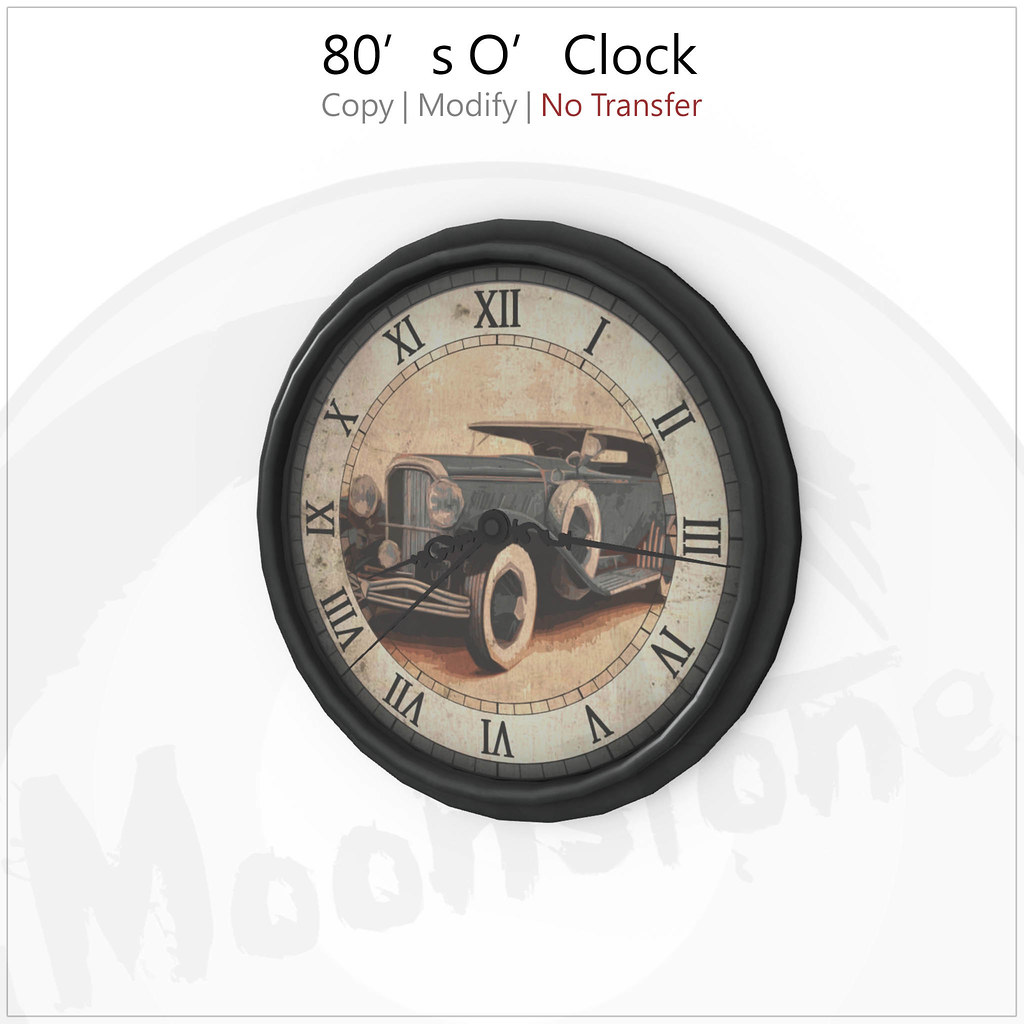The image features a computer-generated clock positioned on a white background, which is subtly overlaid with a large white watermark that curves around the top and bears the faint imprint of the word "Moonstone" at the bottom. At the top of the image, the text "80: S0 o'clock" is displayed, followed by the labels "copy, modify, no transfer" beneath it.

The clock itself, framed with a black rim and displaying minor imperfections and artifacts, surrounds a central antique-style illustration. The round face of the clock is adorned with Roman numerals from I to XII. Within the numerals, an intricate and somewhat modern painting of an early 20th-century grey automobile is situated, facing left with visible bumpers and headlights. The lower and upper portions of the clock's background exhibit a light brownish-beige hue.

The clock's hands are distinct and detailed: the black minute hand points to 3, the shorter black hour hand rests on 8, and an additional tiny silver hand indicates 9, completing the intricate and visually engaging composition.